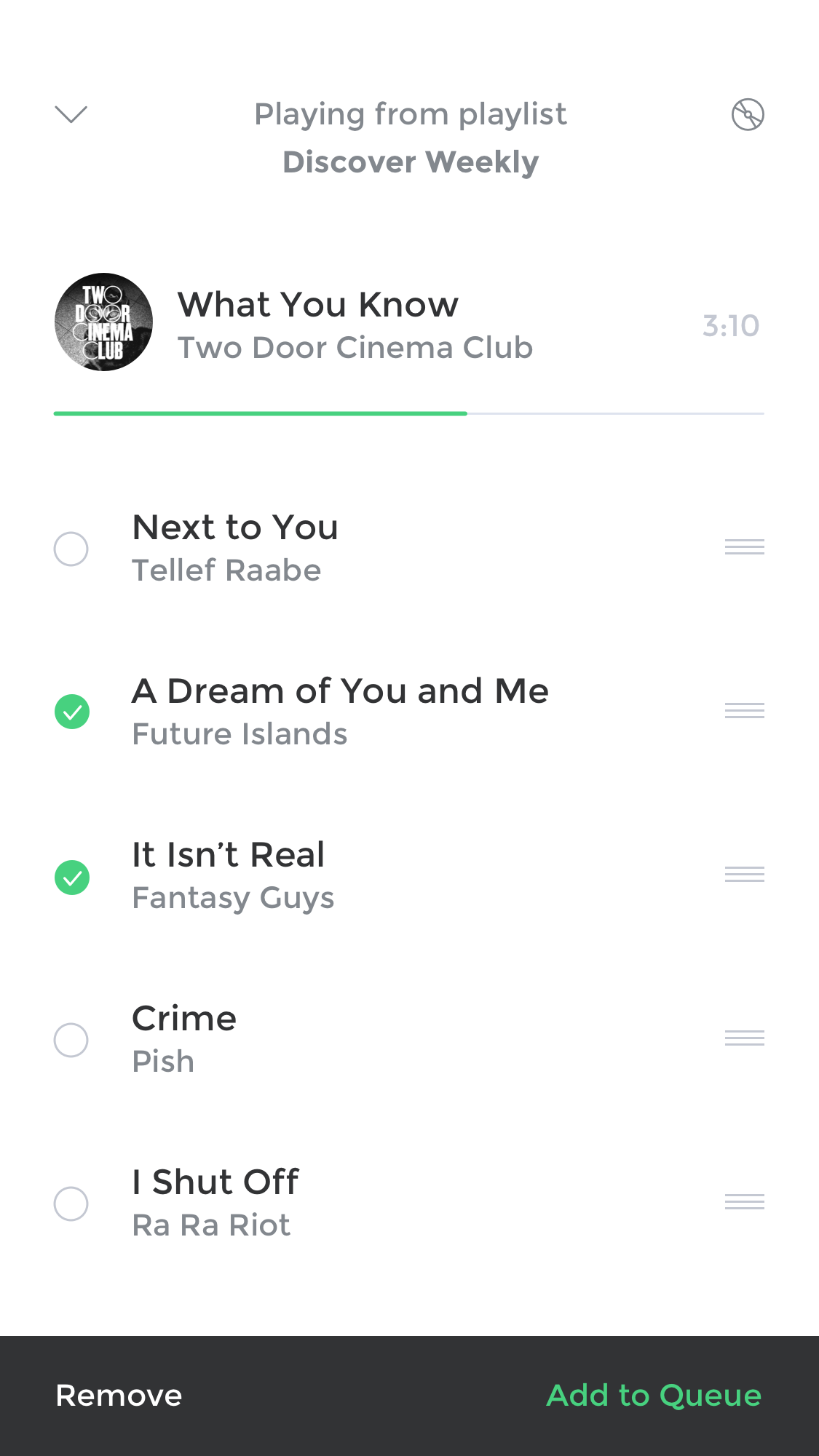Here's a cleaned-up and detailed descriptive caption:

---

This screenshot captures an interface from a smartphone or tablet, showcasing a music streaming app. The top section features a gray bar with a downward arrow and the text "Playing from Playlist" on the right side. Below this, the playlist title "Discover Weekly" is displayed in bold, darker gray text. To the far right is an icon resembling a Pokéball—a circle with a smaller circle inside intersected by an X shape.

Descending further, there is an album cover depicted as a dark gray circle with black bands at the edges, featuring white text with small icon-like bubbles. It reads "Two Door Cinema Club," and to its right, the song title "What You Know" is boldly displayed in black, followed by "Two Door Cinema Club" in dark gray. A timestamp reads "3:10" with no AM or PM indication, and beneath it, a progress bar starts as dark green and transitions to gray midway across.

Below the progress bar, there are bulleted playlists items, with some items selected and others not. Each item starts with bold black text, followed by a gray description. The selected items have a white circle with a gray border, which turns green with a white checkmark when selected. Here are the detailed bullet points:

1. **Next to You**  
   Tellef Raabe

2. **This is a Dream of You and Me** (selected)  
   Future Islands

3. **It Isn't Real**  
   Fantasy Guides

4. **Crime**  
   PISH

5. **I Shut Off**  
   Ra Ra Riot

To the right of each bullet point is an icon resembling a keyboard or three horizontal gray lines.

At the bottom of the screen, a black bezel features two options: "Remove" in white text on the left, and "Add to Queue" as a hyperlink in dark green on the right.